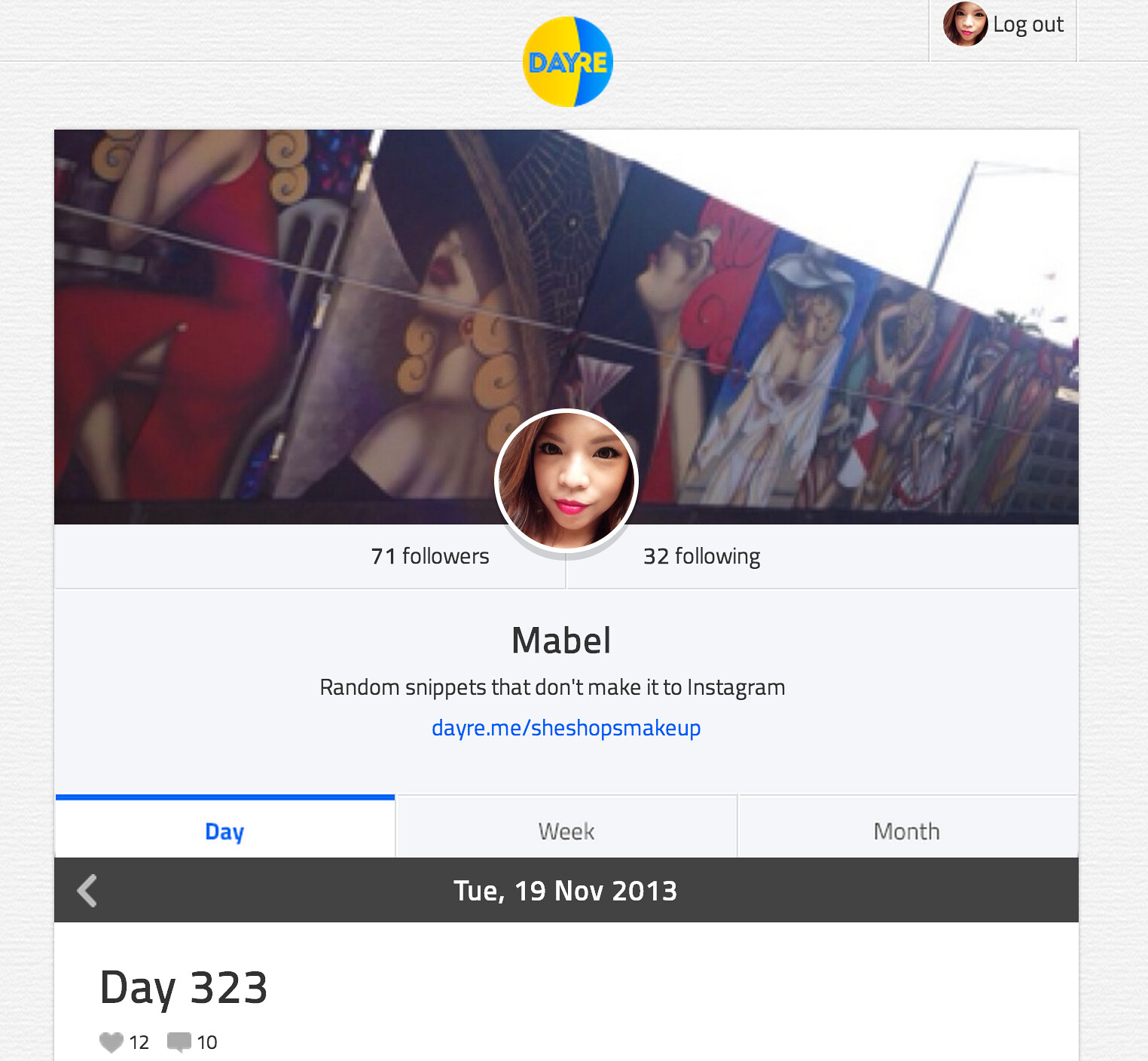The image is a detailed screenshot of a social media website called Dayer, dated Tuesday, November 19, 2013. At the top-center of the screen, the Dayer logo features "D-A-Y" in blue on a yellow background, and "R-E" in yellow on a blue background. On the top-right corner, there’s a small circle profile picture of a young Asian girl in her early 20s. She has long brown hair, bright red lipstick, and dark eyes, with the word "Logout" beside it.

Beneath the logo, there’s a rectangular banner displaying abstract artwork of women dressed in fancy clothes along a fence. In the middle of this banner is a small, repeated profile picture of the same girl. Under this, to the left, it shows "71 followers" and to the right, it says "32 following." The profile name "Mabel" is written below this, accompanied by the tagline "Random snippets that don't make it to Instagram," and the website URL "dayer.me/seshopsmakeup."

At the bottom of the screenshot are three navigational buttons labeled "day," "week," and "month," with the date "Tuesday, 19th of November, 2013" and the text "day 323" inscribed beneath them. The post has 12 likes.